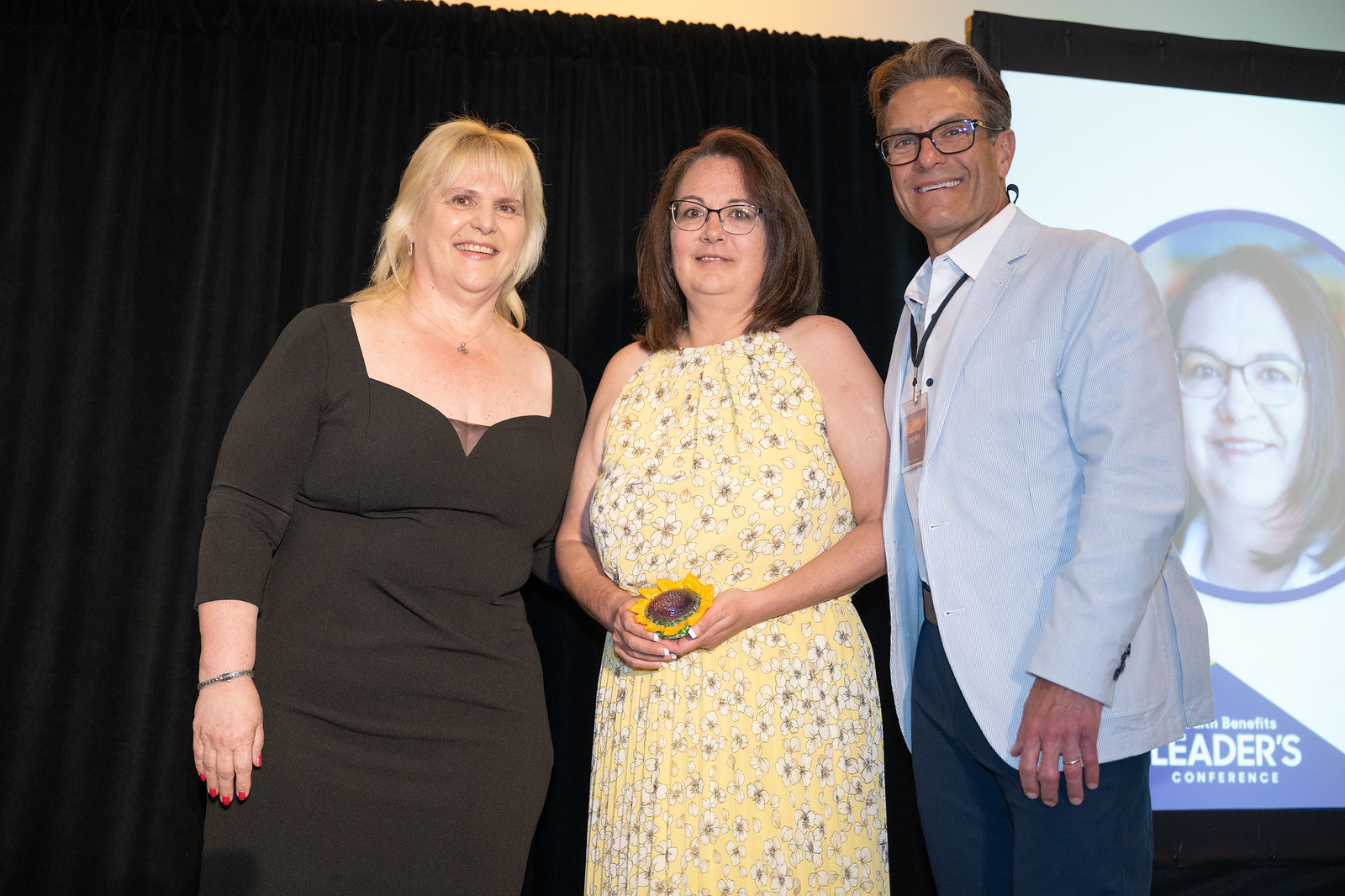This is an indoor image of three Caucasian people standing at the front of a stage, smiling down at the camera. They are illuminated against a backdrop that includes a black curtain and a screen displaying a picture of the woman in the center, labeled with "Leaders Conference."

The woman in the middle of the photo, who appears to have won an award, has shoulder-length brown hair and is wearing glasses and a sleeveless yellow floral dress. She is holding a ceramic trophy designed to resemble a sunflower, painted yellow with a brownish center.

To her left stands a blonde woman in a black dress, accessorized with a bracelet and red painted nails. To the award-winner's right is a man appearing to be around 50 years old, with brown hair combed back, wearing a light blue business jacket over a white collared shirt, and brown-framed glasses. He has a name tag hanging from his neck and is dressed in blue jeans.

Overall, the scene captures a celebratory moment at what appears to be a leaders' conference, with the central figure being recognized for her achievements.